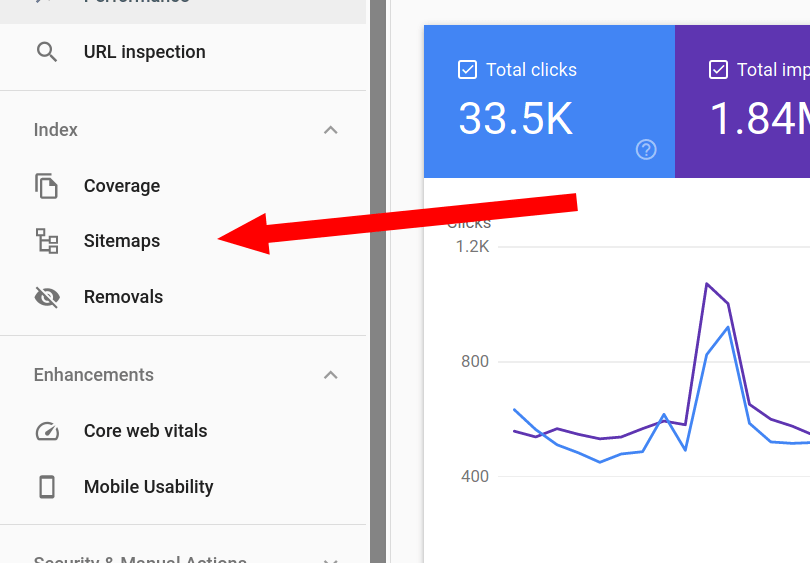The provided image is a screenshot capturing a partial view of a website, giving insight into its interface and functionality. The screenshot is divided into two distinct sections.

On the left side, there is a prominent gray banner extending vertically, suggesting a navigation or menu panel. Within this banner, a darker gray vertical line further segments the area. This section presents several menu options, indicating more content extends beyond the visible portion.

At the top of the gray banner, we see the "URL inspection" option, identified by a corresponding search icon on its left. Below this, a thin gray line separates the top option from the subsequent section, which lists three sub-options under the expanded "Index" section: "Coverage," "Sitemaps," and "Removals," each accompanied by a dedicated icon to their left. Following another thin gray line, there's an "Enhancements" section presented with options to expand or collapse its contents. Currently expanded, it displays "Core Web Vitals" and "Mobile Usability," again with small icons beside each. Finally, the bottom part of the banner is cut off, suggesting additional options are present but not visible in this snippet.

On the right side of the screenshot, the top right corner showcases parts of a dashboard with analytical data. A prominent blue box labeled "Total clicks" indicates a value of 33.5K. Adjacent to this, a partially visible purple box labeled "Total something" hints at additional data. Below the "Total clicks" box, a chart visualizes clickable data trends, featuring blue and purple lines to distinguish between different datasets. Notably, a red arrow, added as an annotation, points from beneath the "Total clicks" box towards the "Sitemaps" section on the left, likely emphasizing a connection or directing attention there.

Overall, this detailed screenshot offers a glimpse into a website's navigation structure and a portion of its analytical dashboard.